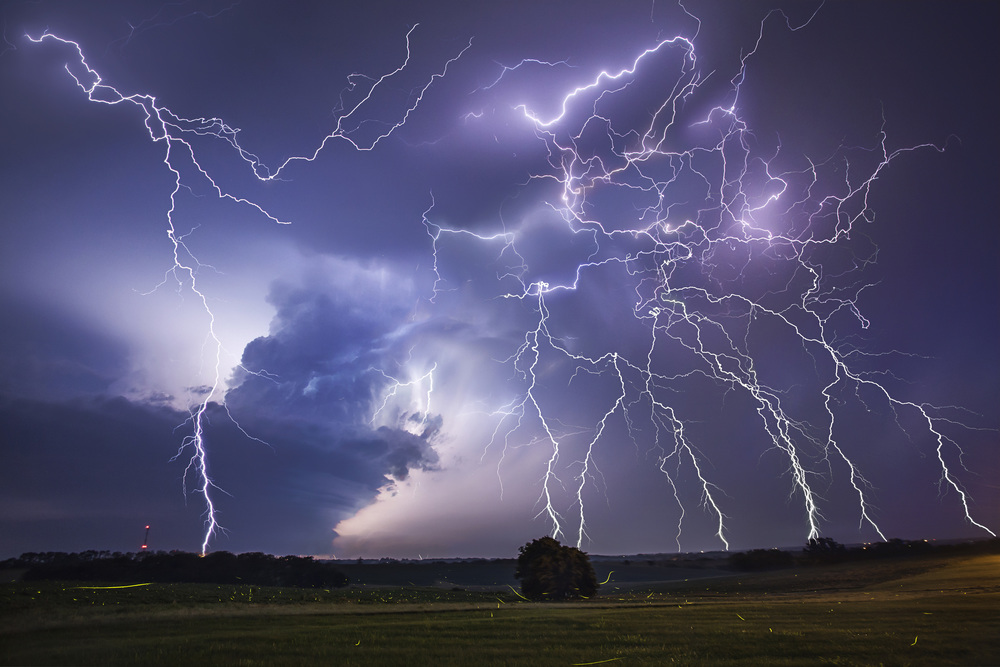The image captures a dramatic countryside thunderstorm with a sky dominated by dark, turbulent clouds in shades of deep blue, purple, and black. Multiple lightning bolts, ranging in color from bright white to white-blue and even purplish hues, streak across the sky, creating an electrifying spectacle. The right side of the image is particularly vibrant with a higher concentration of lightning connecting to the ground. One significant lightning bolt stands out on the left side. The landscape below features a large, lush green field dotted with trees—more densely clustered on the left side, with sparse trees on the right. As the storm unfolds, the fading daylight and the onset of night add to the scene's intensity, with ominous dark clouds obscuring the sun. Some details in the landscape include a crop-filled field, a prominent brown bush with green vines in the middle, and a tower with red lights in the distance on the left. The vast, flat terrain and the stormy sky create a striking contrast, enhancing the overall dramatic effect of the scene.